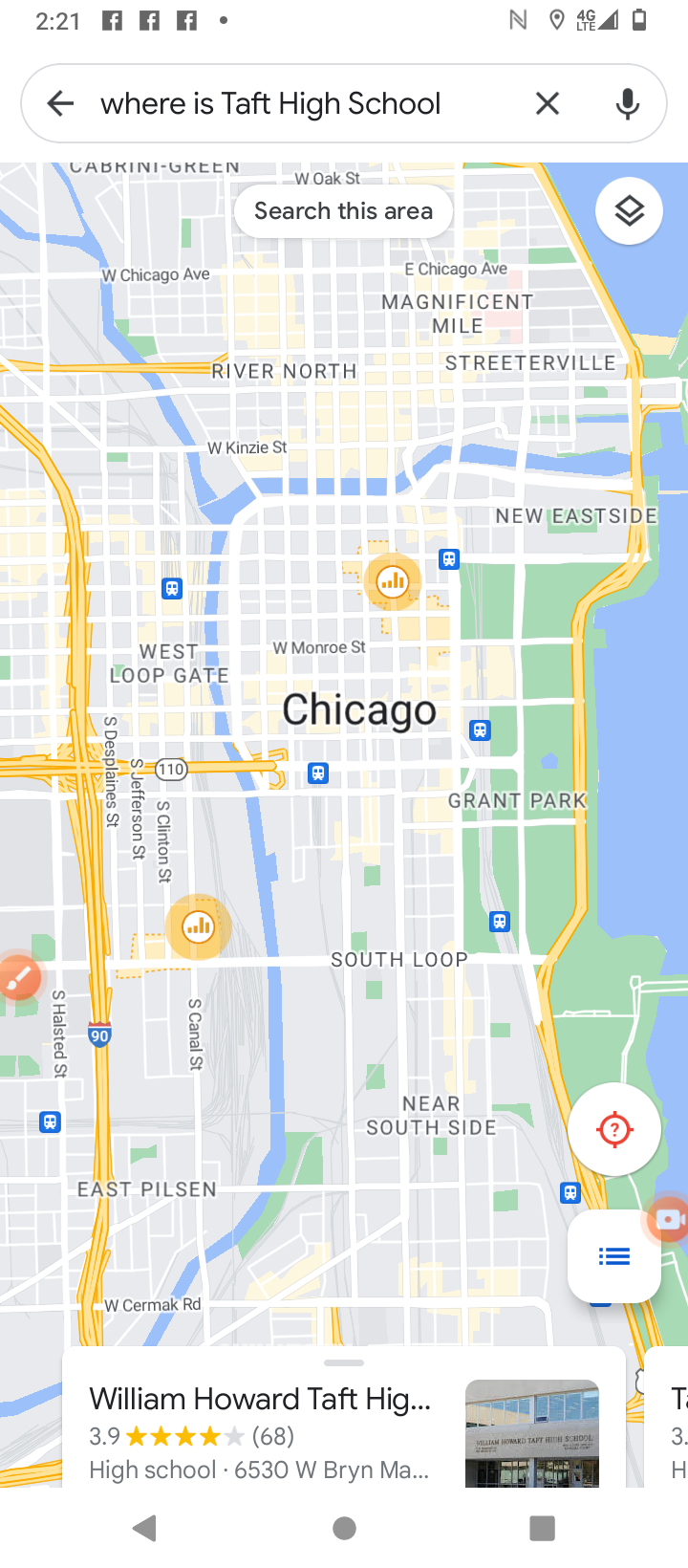The image displays the screen of a smartphone, which could also be a tablet based on its shape, but more likely appears to be a smartphone given the displayed indicators and designations. At the top of the screen, a battery strength indicator, 4G LTE symbol, and a signal strength icon in the form of a triangle are visible. The time shown is 2:21.

Prominently, the image highlights a map of Chicago, featuring key areas such as Grant Park, Near South Side, South Loop, West Loop Gate, East Pilsen, Streeterville, and Magnificent Mile. Major highways like I-90, cutting through the city, and Highway 110, running east-west and connecting with I-90, are clearly marked.

Additional elements include icons for Facebook buttons and a "Quick Connects" feature. At the bottom of the screen, there is a quick link to William Howard Taft High School, showing ratings and the number of ratings given. The detailed map focuses on central Chicago, particularly highlighting the Loop and downtown areas.